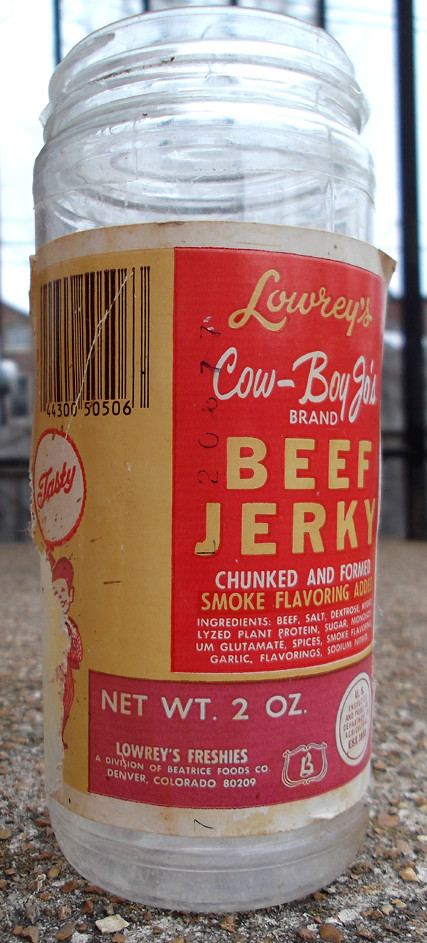The image features a can of Lowry's Cowboy Joe's Brand Beef Jerky, labeled as "chunked and formed" with added smoke flavoring. The net weight of the product is 2 ounces. The can bears the "Lowry's Freshies" branding, indicating it is a division of Beecher's Foods Company based in Denver, Colorado, with the ZIP code 80209. On the bottom right of the label, there is a distinct logo featuring a "B" in black or red. The upper left section of the label displays the word "Tasty" in yellow. Additionally, the barcode number 4430050506 is visible. The can itself is white, housing the label, which wraps around the container, making it appear consistent with other packaging for this type of product.